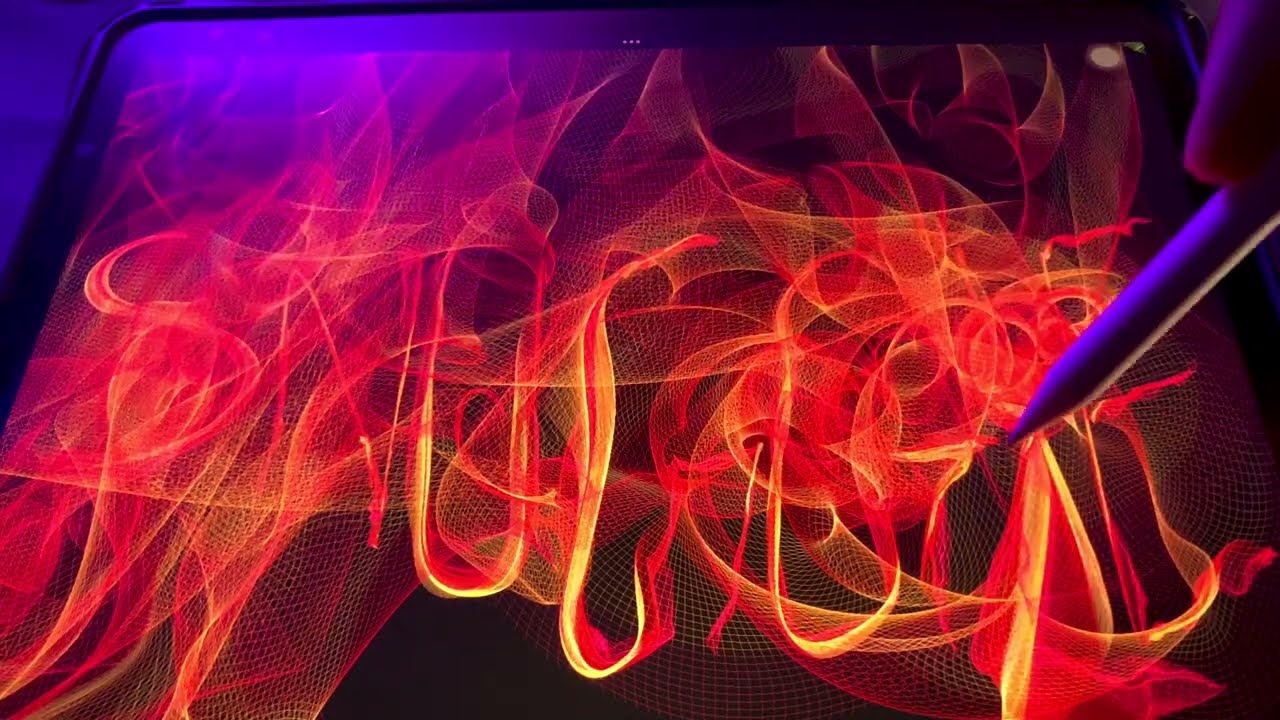The image shows a person using a stylus on a tablet that is propped up on a table. The hand holding the stylus is positioned on the right side of the image, actively engaged in digital drawing. The screen, which has a black background, features a vibrant, neon-like graphic with letters and flames. The letters, which appear to spell a word starting with 'S' followed by 'N' and 'O', are partially obscured by dynamic strokes of fiery red, yellow, and orange lines. These lines give the impression of 3D flames or neon lights. The top of the screen displays three dots, suggesting the user interface of the drawing app. Additionally, a purple light subtly illuminates the scene, adding to the digital art's vividness. The drawing’s lower part is marked by U-shaped yellow designs, enhancing the fiery effect of the overall composition.